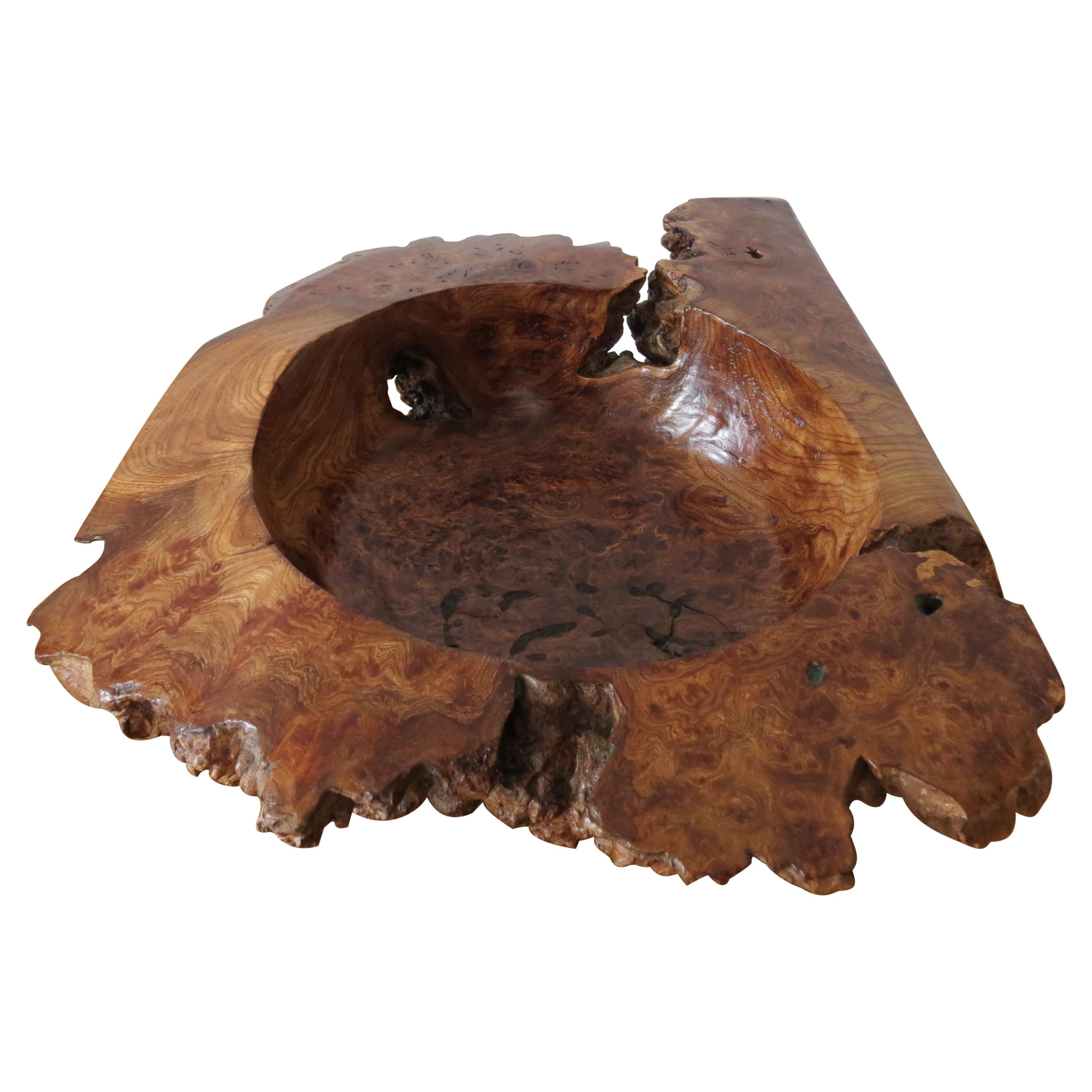This image captures a remarkable wooden sculpture, resembling a large, handcrafted bowl. Made from a piece of varnished wood, likely a section of a tree stump, it boasts a rough, natural exterior as though it was shaped by nature or a saw. The interior, in contrast, is smoothly hollowed out to form a bowl-like shape, highlighting the artisan's skill. The polished surface enhances its shiny appearance, while two small natural holes within the bowl reflect the authenticity of the wood. Despite its bowl shape, it serves more as a sculptural piece than a functional vessel, with subtle edges that don’t meet completely at the back, adding to its unique aesthetic.